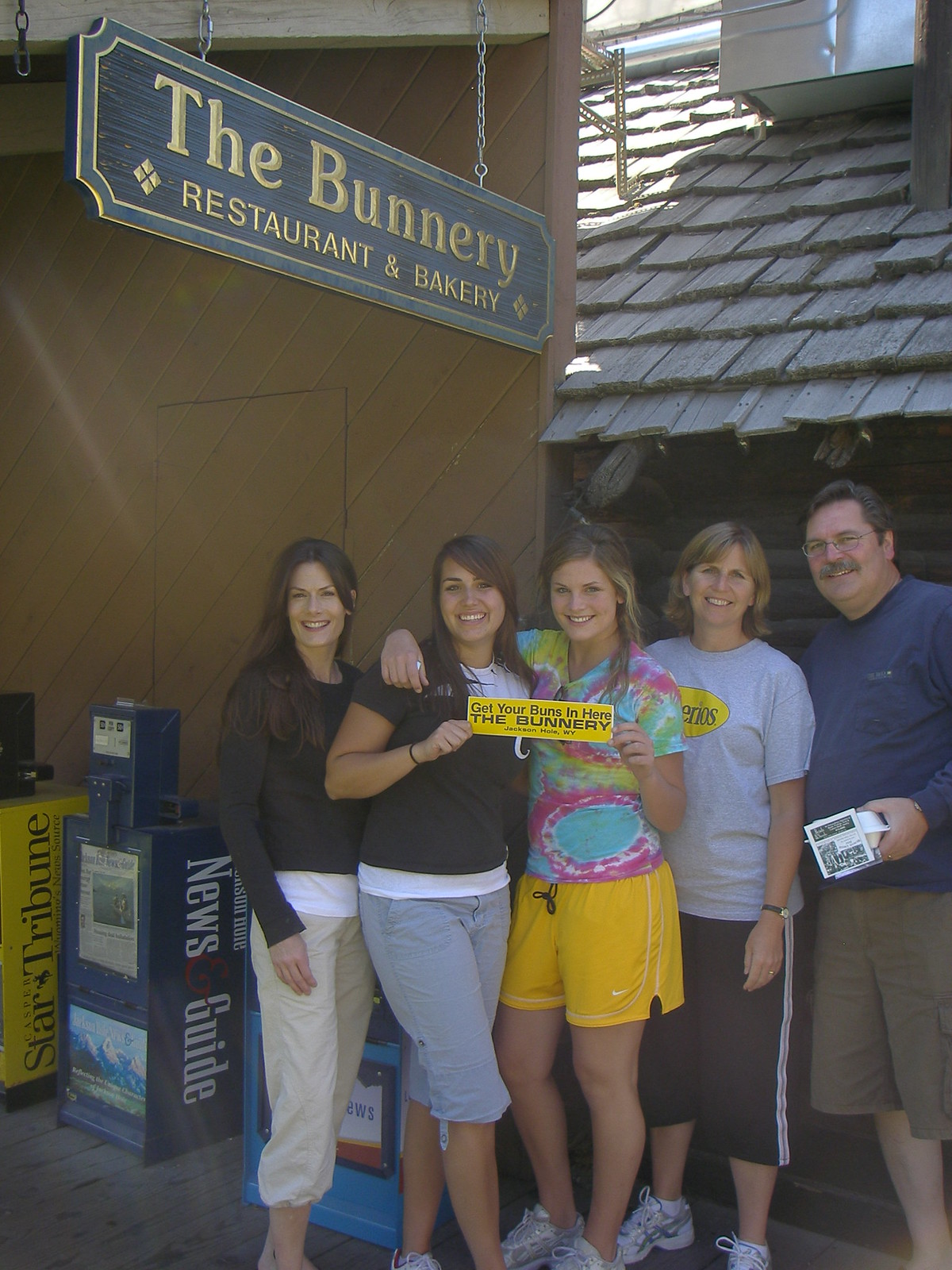This outdoor image captures a bright, midday scene in front of "The Bunnery Restaurant and Bakery," a charming establishment with a gabled roof and mustard-colored walls. The main sign, suspended by chains, features golden text on a blue background, prominently displaying the restaurant's name. In the foreground, five individuals—a man and four women—stand posed and smiling for the camera. The man, likely in his fifties, sports a blue sweatshirt, khaki pants, glasses, and a slightly gray mustache. To his left, a woman of similar age, with blonde hair, is dressed in a white and grey t-shirt and capri pants with a dark, white stripe. Next to her, a young blonde woman in her twenties wears a tie-dyed pink and green shirt, yellow shorts, and white sneakers. Her arm is around another woman clad in a black sweater and gray capris. The final person on the left, a young woman with a ring, wears khaki pants and a black shirt, resting her hand on the middle woman. The group is holding a bright yellow sign with bold black lettering that reads, "Get Your Buns In Here, The Bunnery." In the left corner of the image, there are a couple of newspaper boxes marked "Star Tribune News Guide," adding a touch of everyday life to this friendly and inviting scene.